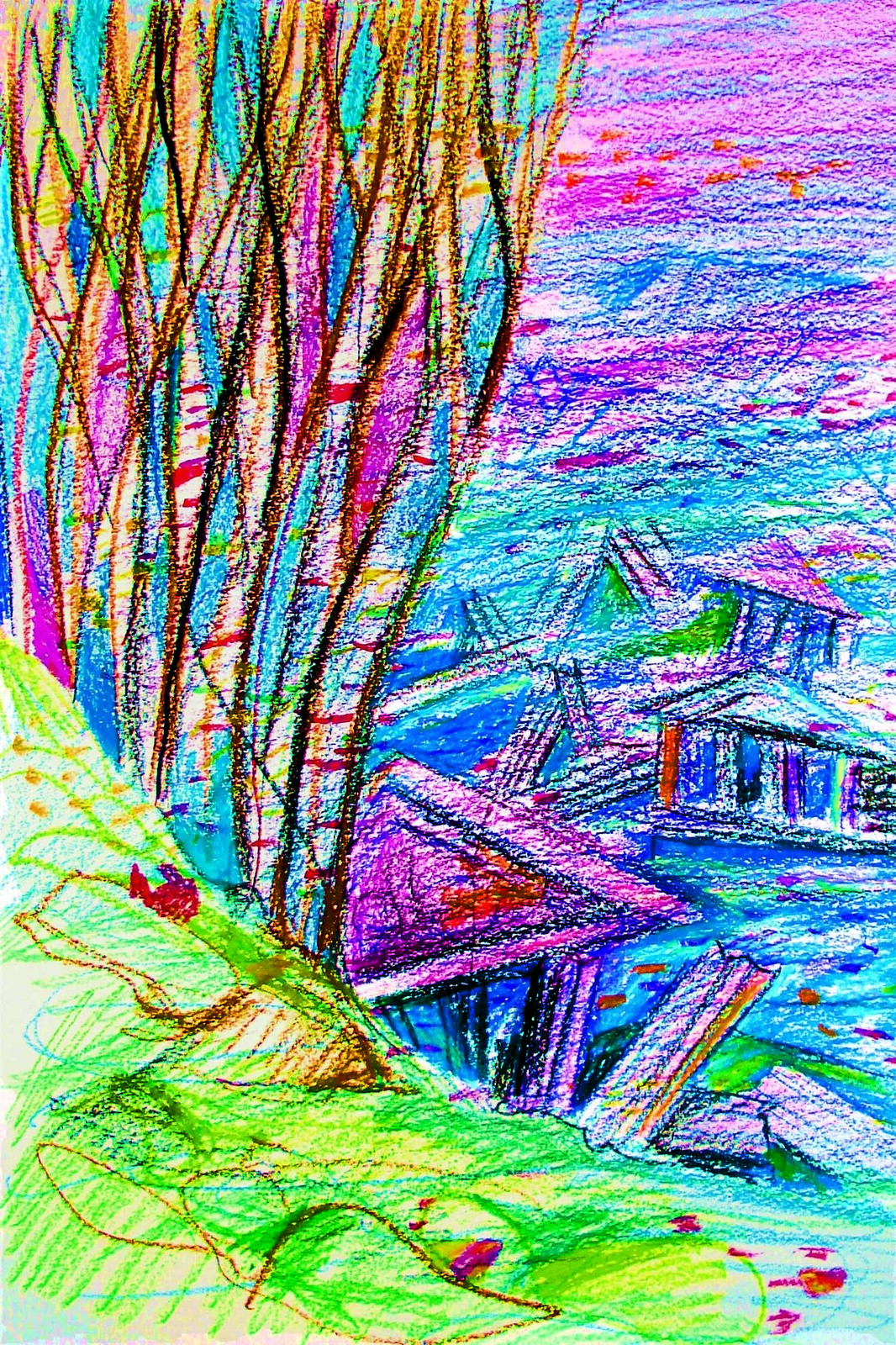This is a detailed and expressive crayon sketch depicting a devastating scene of a natural disaster, a flood. The foreground showcases a green, bumpy hillside or cliff adorned with young trees and bushes. Scattered among the green are some buildings, distinguishable by their purple roofs, precariously situated beneath the cliff, one appearing miraculously intact amidst the chaos. The hillside gives way to a turbulent river, with shades of angry blue and disturbed currents illustrating the floodwater. Broken pieces of piers and docks, possibly from a marina, float amidst the wreckage, signifying the force of the flood. The riverbank is depicted with a raw feeling of destruction, with homes partially submerged and their windows eerily peeking through the water, surrounded by debris. A mix of colors—blues, purples, and pinks—distorts the landscape further, capturing the surreal and overwhelming nature of the flood. The scene, while chaotic, is framed by the ominous blend of colors in the upper part of the image, resembling a sunset but tinted with distress, adding to the emotional weight and vivid depiction of this catastrophic event.